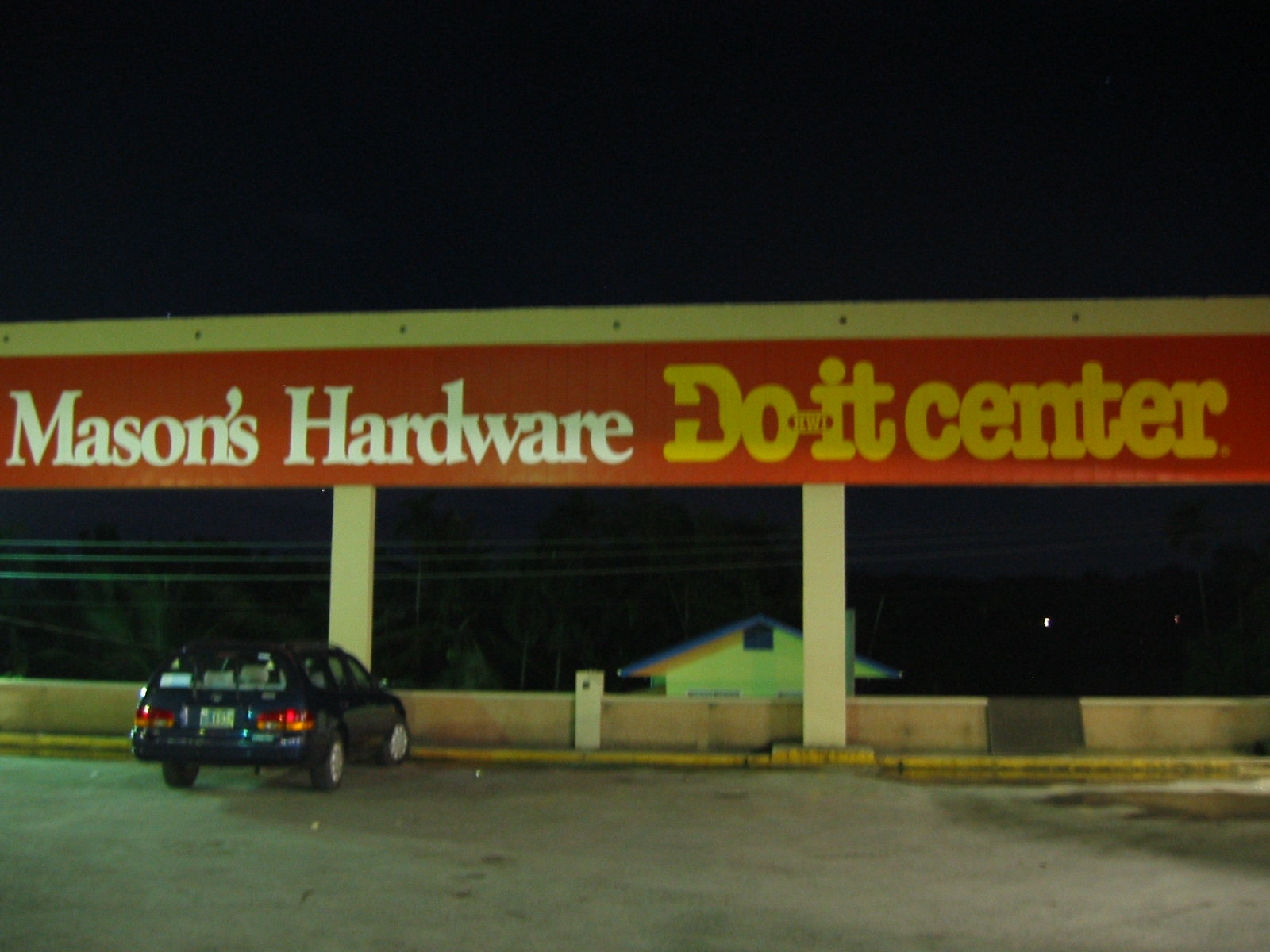This nighttime photograph, with a horizontal orientation, captures a scene in a parking lot. The inky black sky suggests the late hour. Dominating the center of the frame is a large, prominent sign that reads, "Mason's Hardware Dewitt Center." The words "Mason's Hardware" are displayed in bright white letters, while "Dewitt Center" is highlighted in yellow, all set against a bold red background. The sign is framed in what appears to be natural wood, though the dim lighting makes this detail somewhat ambiguous.

In the background, a small house is visible beyond the sign, adding a touch of domesticity to the otherwise commercial setting. Below the sign is a low concrete divider, marking the boundary of the parking area. To the left side of the frame, a single vehicle—a station wagon or hatchback—is parked diagonally with its rear end facing the viewer. The concrete end of the sidewalk, painted yellow, is visible and serves as a cue for where vehicles should stop when parking. Hanging beneath the Mason's Hardware Dewitt Center sign are a series of telephone lines, adding to the urban feel of the image. The scene likely represents a big-box store's parking lot, captured under the cloak of night.